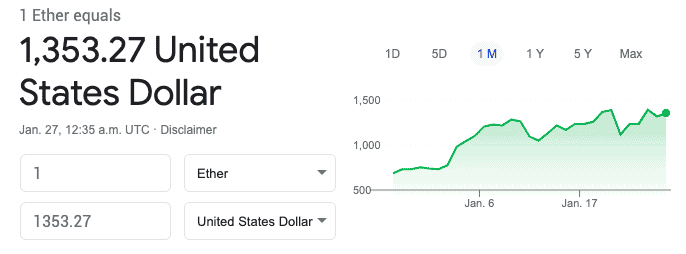Screenshot Details of Ethereum's Value Against USD on a Financial Chart

The image is a screenshot featuring a white background with various financial details prominently displayed. On the left side, the text indicates that "1 Ether equals $1,353.27 USD" as of January 27, at 12:35 AM UTC, with a disclaimer noted below. A series of boxes are shown: one with the number "1," another with "1,353.27," one labeled "Ether" featuring a drop-down arrow, and another labeled "United States dollar" with a drop-down arrow.

To the right of these boxes is a financial graph displaying a green, spiky line trending steadily upwards. Above the graph are time selections: 1D, 5D, 1M (which is selected), 1Y, 5Y, and MAX. The right side of the graph includes numerical markers: 1500, 1000, and 500, indicating price levels. Below the graph, date markers are present, showing "January 6th" and "January 17th," with a notable green dot at the graph's endpoint.

The image is wider than it is tall and contains purely graphical and text elements, devoid of any photographic components. There are no people, animals, plants, flowers, trees, automobiles, or motorcycles depicted in this image.